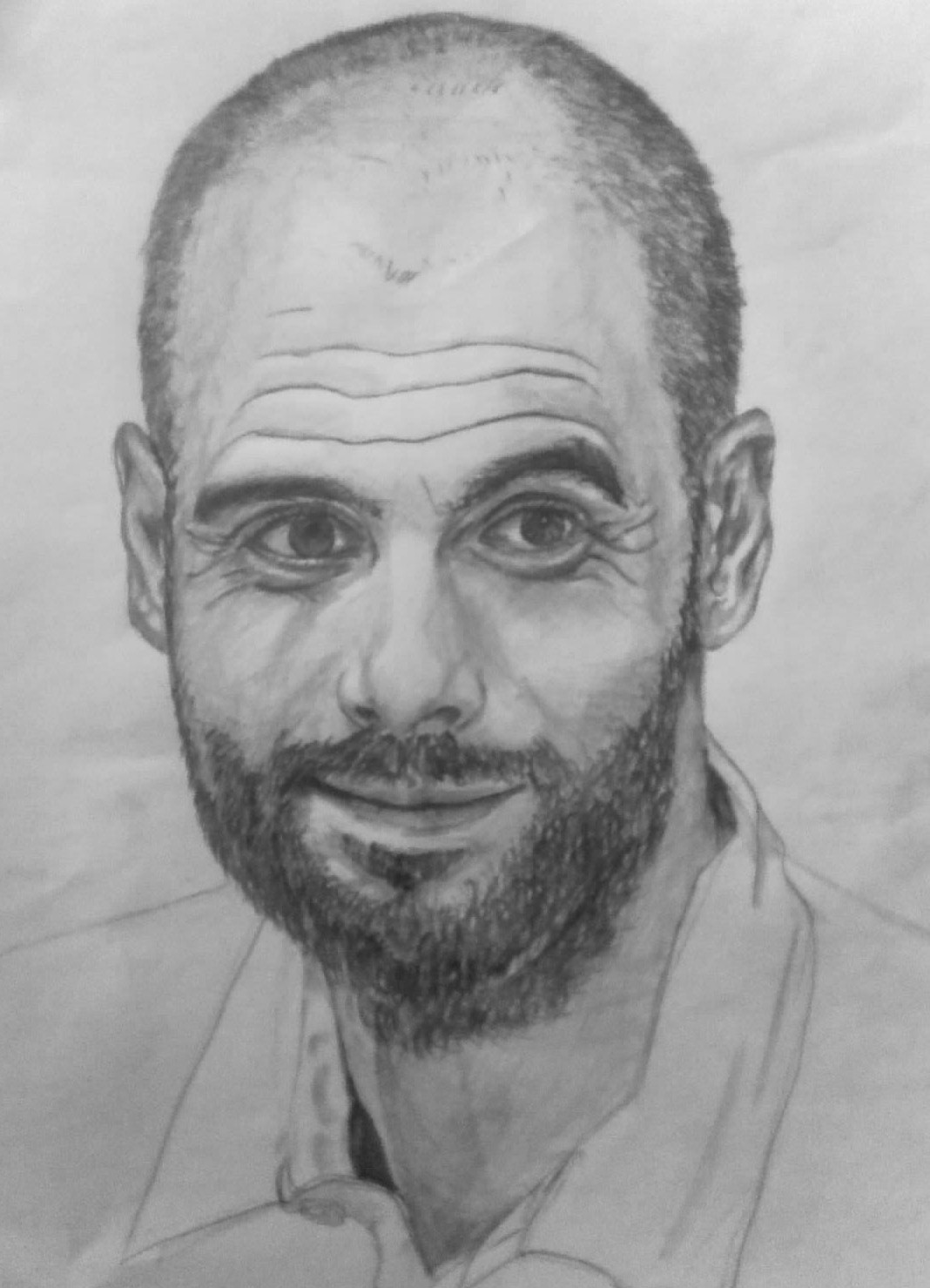This is a monochrome pencil drawing of a gentleman, meticulously sketched on white paper. The man is balding, with a receding hairline and short, buzzed hair remaining at the crown and around his ears, tapering into sideburns that seamlessly blend into a well-groomed beard and goatee mustache. He is depicted wearing a white-collared dress shirt. His face features intense shading and intricate details that bring out a dimensional quality. Notable facial details include deep smile lines and pronounced wrinkles: three thick lines cross his forehead, with an additional smaller one on the right, and crow's feet accentuate his crinkled eyes, which are framed by thick, bushy eyebrows. His pupils are heavily shaded, and the intricate work around his lips, using dark and light gray tones, adds further depth. The left ear is slightly larger than the right, enhancing the asymmetry and realism of the portrait. The entire composition, from his smirk to the texture of his facial hair, is rendered in varying shades of black, white, and gray, presenting a lifelike and expressive portrayal of a man smiling.